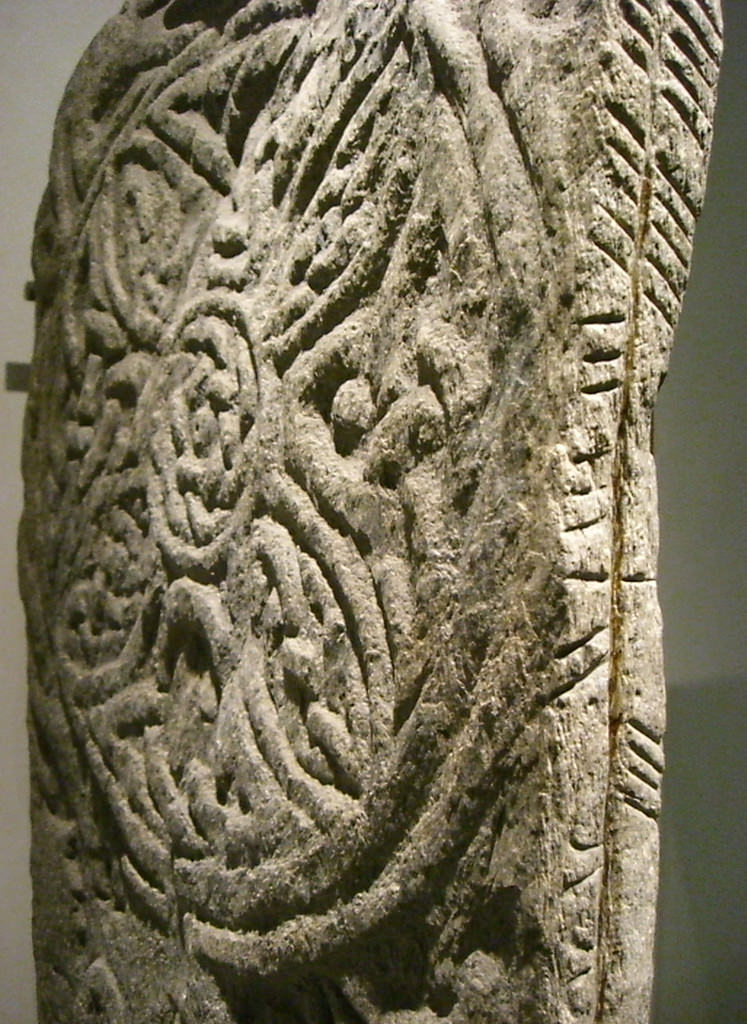A color photograph taken indoors in portrait mode captures a large rectangular stone with the top and bottom edges cropped off. The stone is slightly tilted to the left and features rough, coarse engravings and textures. Intricate yet unrefined, the carvings display a variety of curved lines, grooves, and shapes. The centerpiece of the stone reveals a circular design, surrounded by the textured landscape. In the foreground, a prominent vertical line runs the full height of the stone, intersected by diagonal lines that traverse its surface.